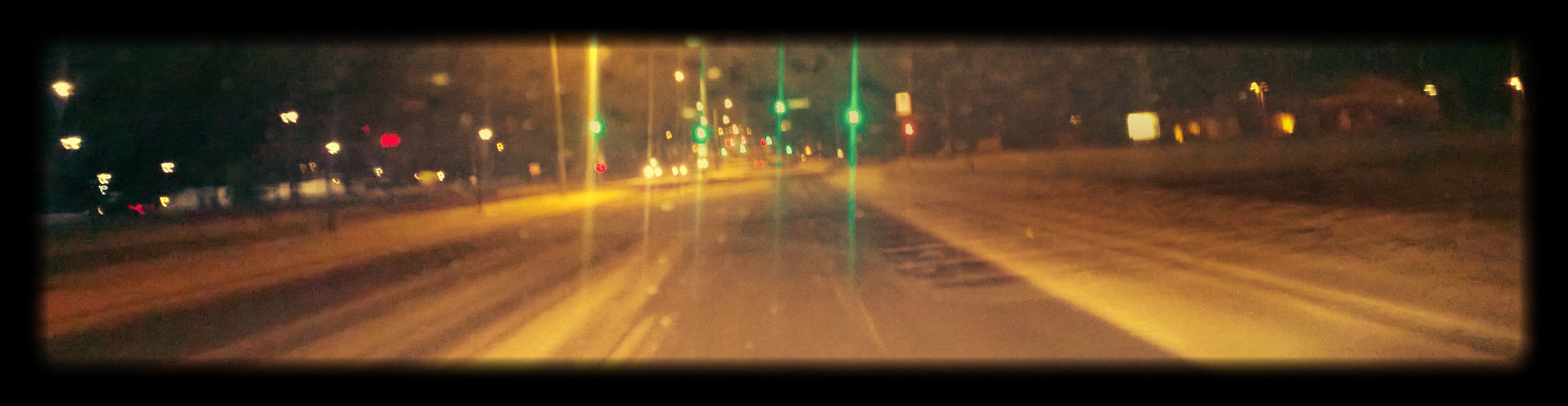Captured after dusk, this image showcases a serene, snow-covered town road. The scene unfolds on a two-lane road where the right lane is clear of snow, providing a navigable path, while the left lane and center median are blanketed in a layer of untouched snow. Snow also covers both shoulders of the road and the adjacent sidewalks, leading to a picturesque landscape.

On the right side, an open field stretches out, dotted with a few trees and flanked by snow-covered grass. In the background, houses are set back from the road, illuminated by distant streetlights that cast a gentle glow across the scene. 

Approaching an intersection, you can see four vibrant green traffic lights beckoning onward movement. The cross signal indicates it's safe to continue straight ahead. A handful of cars are approaching from the opposite direction on this divided road. To the far left, a few neon signs and additional streetlights highlight various buildings, adding a touch of color and life to the tranquil, snowy night.